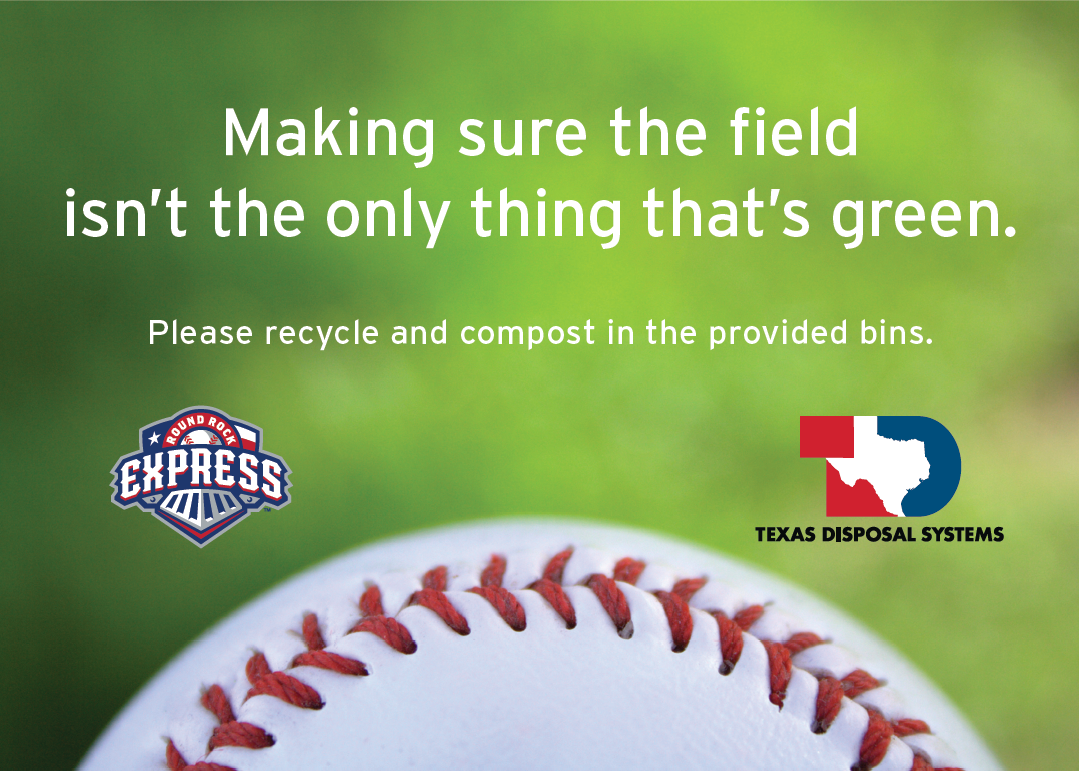This promotional slide features a blurred background that transitions through various shades of green, potentially evoking a grass field. Dominating the bottom third of the image is the top half of a pristine white baseball with prominent red stitching, stretching across the width from the lower right to lower left. Above the baseball on the left side, there is the Round Rock Express logo in red, white, and blue. On the right side, there is the Texas Disposal Systems logo, which incorporates the outline of the state of Texas colored in red and blue. The header, displayed in white text at the top of the image, reads, "Making sure the field isn't the only thing that's green." Just below this, smaller text urges viewers to "Please recycle and compost in the provided bins." The overall tone and imagery emphasize environmental consciousness within the context of baseball.